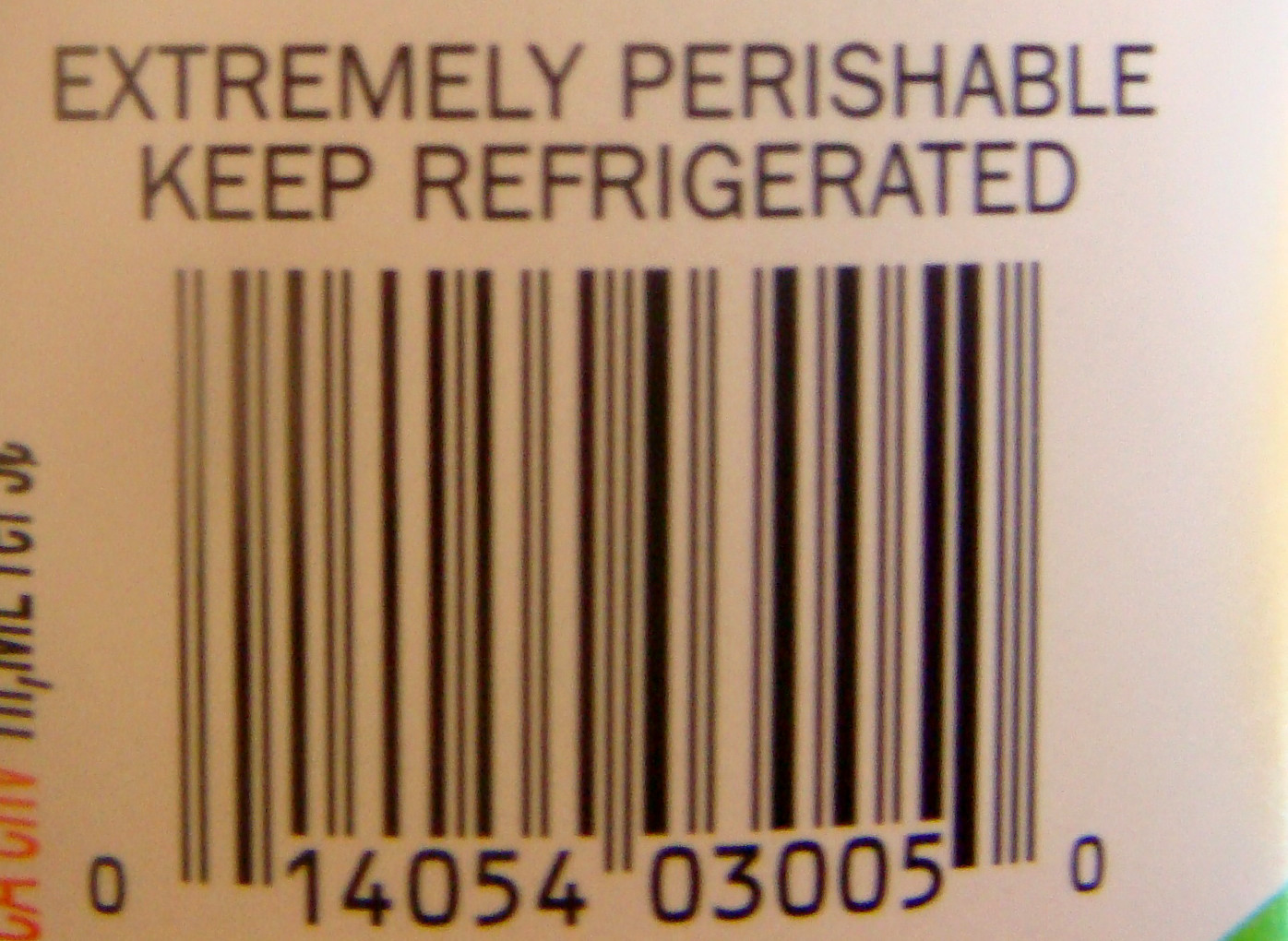A close-up image of a barcode dominates the frame, rendered in stark black and white contrast. The barcode, with its series of vertical black stripes on a white background, features numeric details at the bottom reading "014014054030050." Above the barcode, in bold, capitalized black letters, the words "EXTREMELY PERISHABLE, KEEP REFRIGERATED" are prominently displayed. The lighting in the image is less than ideal, casting uneven shadows across the barcode. A small speck of green is noticeable in the bottom right corner, while a hint of red writing peeks through in the bottom left, adding subtle splashes of color to an otherwise monochromatic scene.